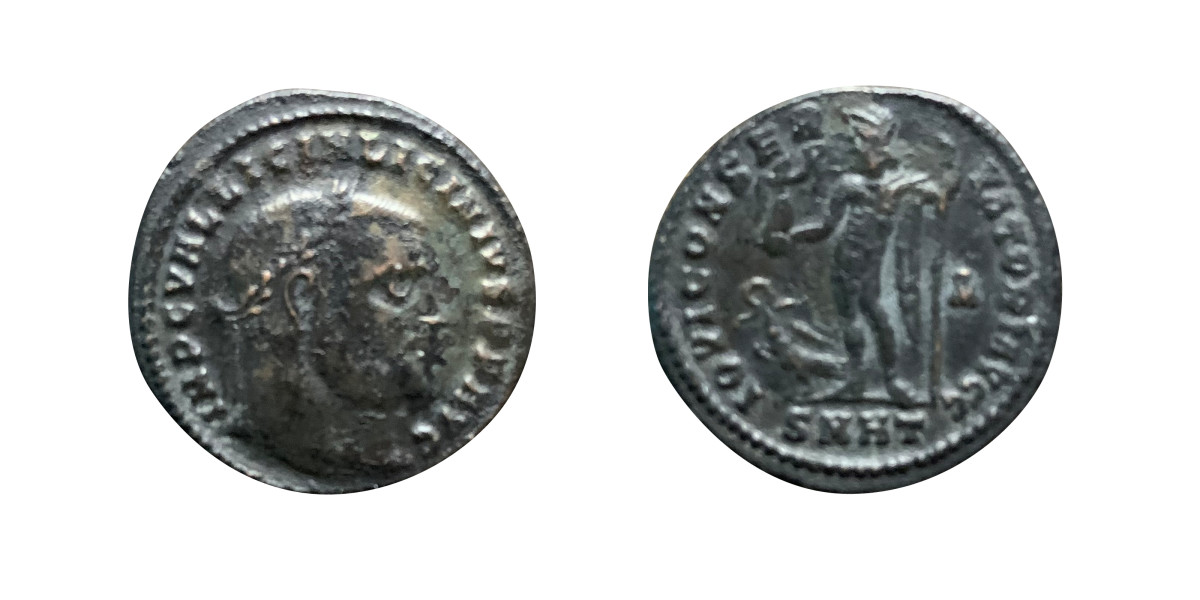This image depicts two ancient coins placed side by side against a stark white background. Both coins, roughly the size of dimes, exhibit considerable age and wear, with one side noticeably more tarnished than the other. The coins appear to be made of silver, though they have developed a brownish patina over time. Both coins feature heavily faded inscriptions along their outer edges, too indistinct to decipher clearly.

The left coin, presumed to be the obverse side, shows a portrait of what appears to be a Roman emperor adorned with a laurel wreath—a symbol of heroism. This side is notably more worn and tarnished. The right coin, likely the reverse side, depicts a figure, possibly a pharaoh or a warrior, standing and holding a staff in his left hand with a helmet on his head. His right hand is extended, holding an unidentifiable object. Both coins are round but irregularly shaped, with ridged edges and varying thickness. Although the inscription "SNHT" is somewhat discernible at the bottom of the right coin, the rest of the text remains illegible, suggesting these ancient artifacts likely originate from a non-English-speaking culture.